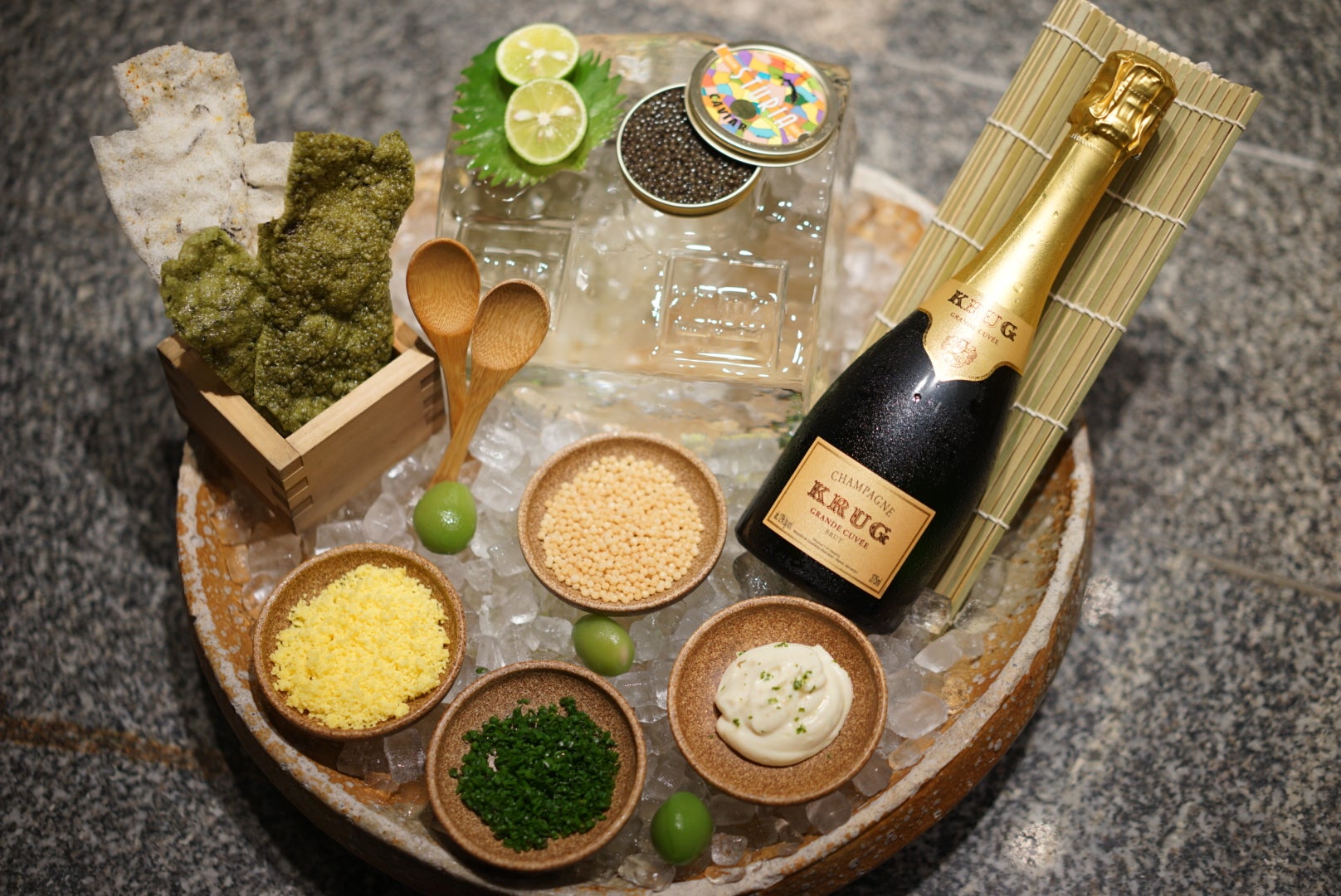This meticulously arranged photograph showcases an elegant wine and snack tray set atop a black and white marble countertop. The main feature is a round brown platter filled with ice, which helps keep a variety of small brown bowls chilled. These bowls contain an assortment of delicacies, including yellow, green, brown, and white food items, likely caviar, seaweed, and cream, along with green olives nestled around the ice. Positioned towards the top right of the image is a prestigious Krug champagne bottle, adorned in its distinctive black and gold label, reclining against a bamboo or straw mat embedded in the ice. Nearby, a square wooden box houses assorted crackers, complementing the sophisticated spread. Additionally, a couple of wooden spoons are strategically placed within the tableau, enhancing the overall presentation of this luxurious and inviting serving arrangement.